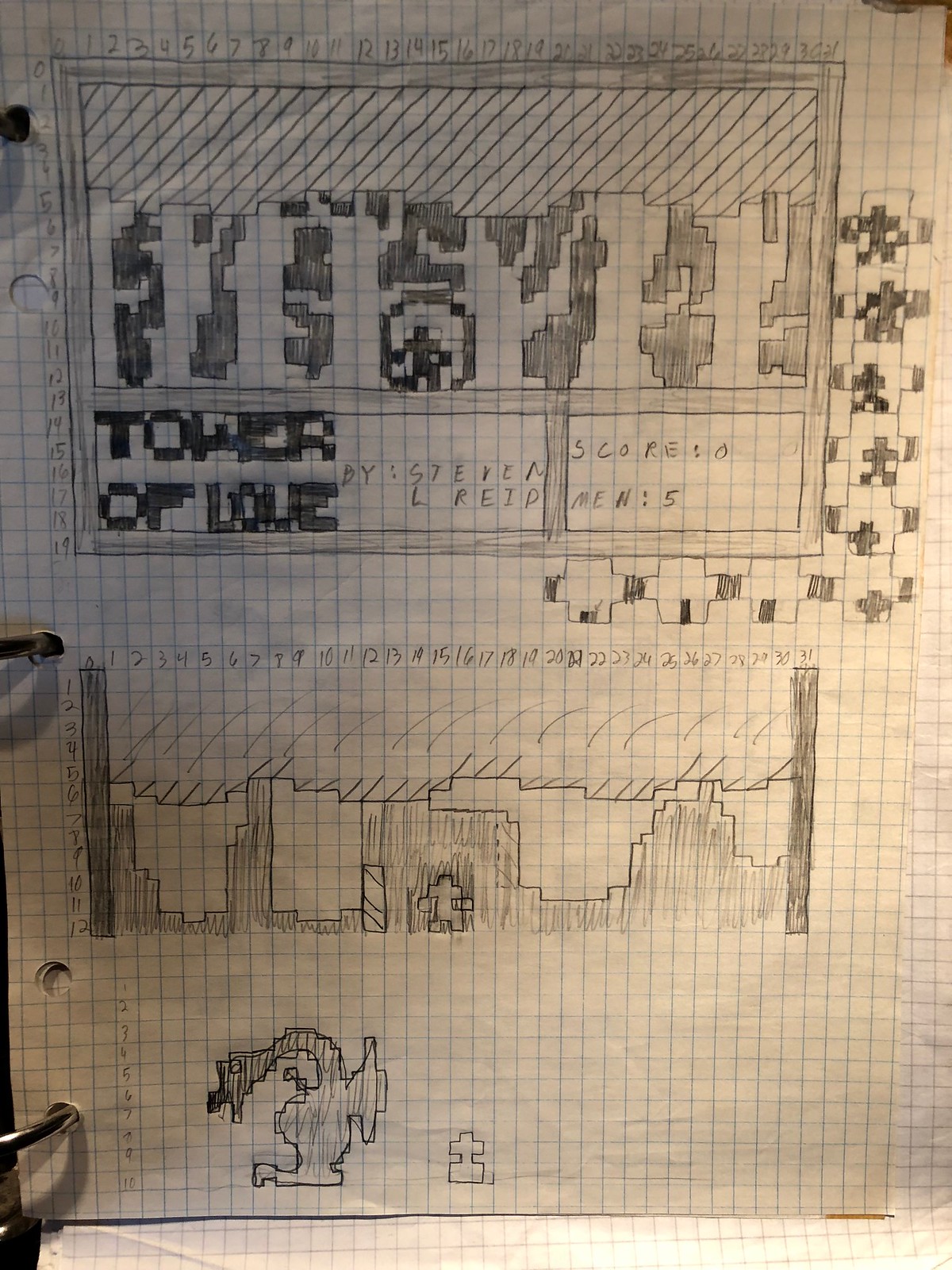The photograph shows a meticulously sketched board game on a sheet of white paper with a grid of small blue squares, viewed from above. The paper is hole-punched along the left-hand side. The game, titled "Tower of Love" by Stephen L. Reid, features two distinctive sections. 

At the top portion, there is a large rectangular area filled with slanted lines and various random patterns created by shading individual squares. This section also includes a maze in the center of the rectangle.

The middle portion showcases arrays of numbers oriented horizontally and vertically, forming a graph-like pattern. Next to this graph, shaded patterns resemble puzzle pieces. Below this section, "Tower of Love" is prominently shaded in, alongside what appears to be the name "Scorpio" and some other indiscernible elements.

The lower part features another similar game. It starts with a sketched image incorporating shapes like a handle, rectangle, circle, long curved line, and a lever on the right-hand side. A chart with shaded areas mimics a graph, with numbers labeled 0 to 19 along one axis and up to 25 along another. Little square-drawn men are placed on the right-hand side, and a score section is noted with "men 5, scorers 0." Both sections include maze-like drawings and shaded puzzles, suggesting a consistent theme across the two games depicted on this detailed blue grid paper.